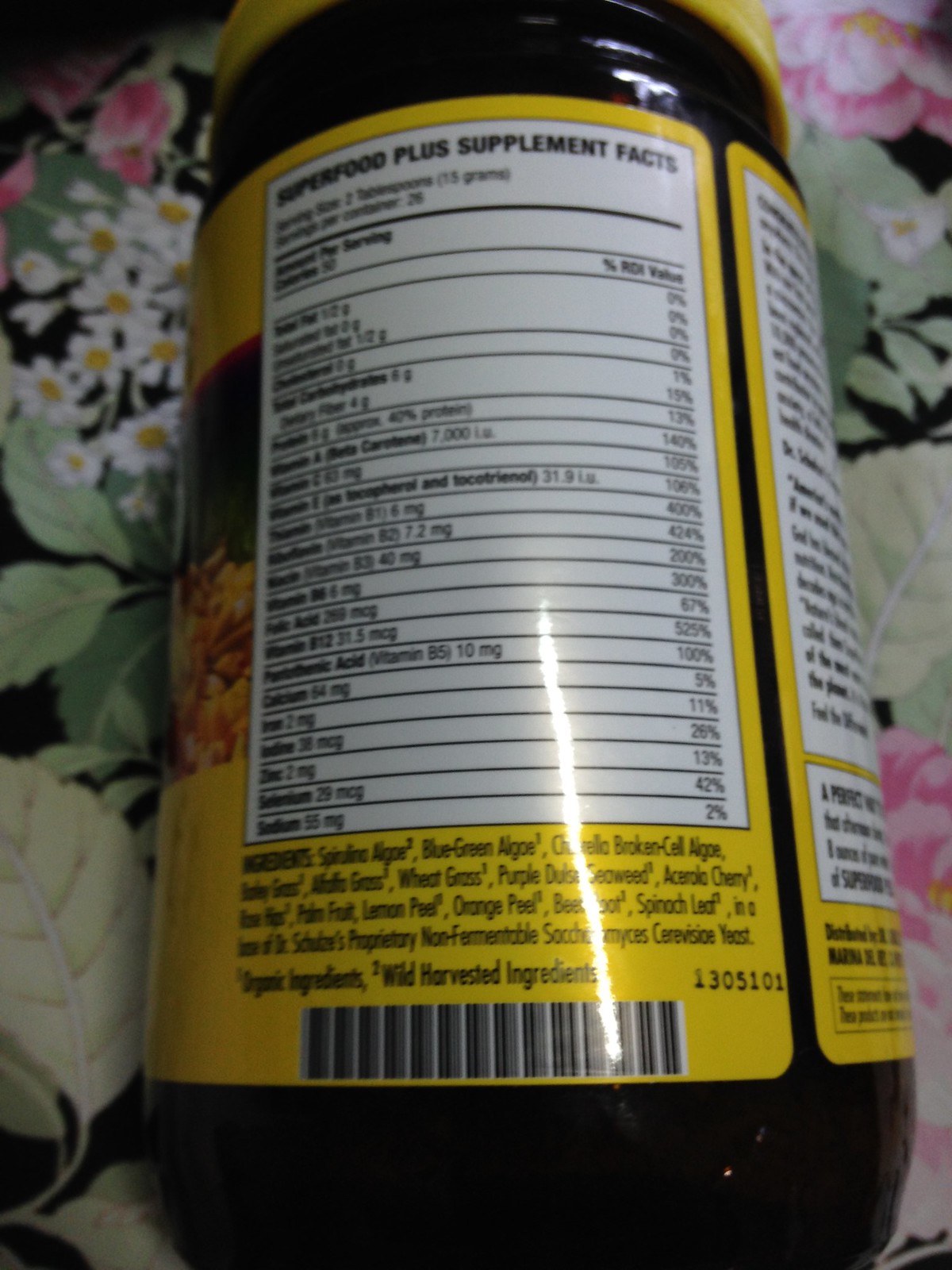This image features the back label of a vitamin supplement bottle. The label is detailed and prominently displays "Superfood Plus Supplement Facts." It specifies that the serving size is two tablespoons and provides detailed nutritional information, including the various vitamins and minerals contained within the supplement. The list of ingredients begins with algae and is followed by green algae and brown algae. The label also appears to mention "purple dulse," although the text is partially obscured. Overall, the label offers comprehensive information about the contents and nutritional benefits of the supplement.